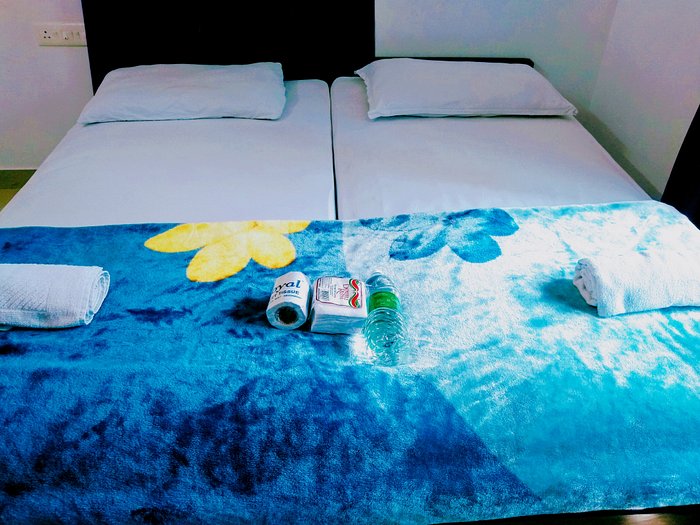This detailed photograph captures an arrangement of two twin-sized beds that have been pushed together to form a larger, king-sized sleeping area. The beds are dressed in simple white sheets with matching white pillowcases. Draped across both beds, approximately halfway down, is a plush floral blue blanket. The blanket displays a striking yellow flower in the center and a blue flower, adding a touch of color to the serene setting. Flanking the blanket, on each side of the beds, are rolled-up white towels. Spanning the middle of the blanket are three items: a bottle of water, a stack of napkins, and a roll of toilet paper still wrapped in its packaging. The background features a white wall with visible switch plates on the upper left side, and a glimpse of dark wood tile in the lower right corner of the image. This carefully detailed setup suggests a pristine, possibly hotel-like environment, inviting and methodically arranged.